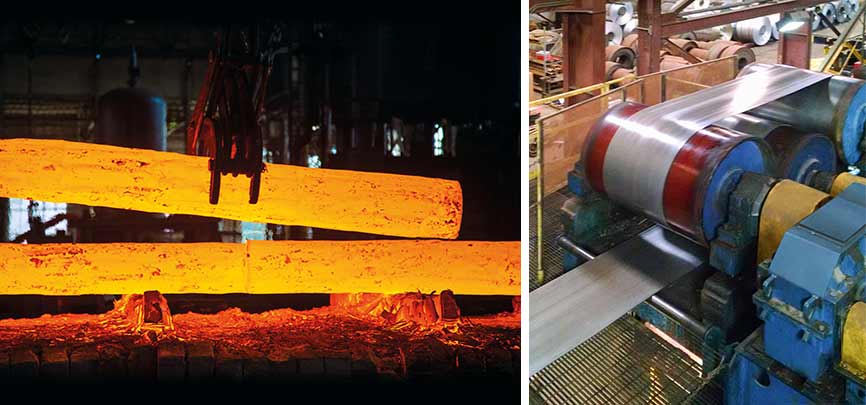The image is divided into two photographs. On the left side, machinery grips and maneuvers two red-hot cylindrical metal pipes, one of which is being placed on top of another, both glowing a bright orange from intense heat. The scene is set within what looks like the interior of a warehouse or industrial setting, where the glowing structures are supported by additional heated metal components. In the background, various industrial pipes and tanks are faintly visible, adding to the complex environment.

On the right side, there is a detailed view of an intricate conveyor belt system. A prominent blue machine with numerous wheels and rollers stretches out a silver material. Among these rollers, one stands out, glowing bright red from the heat and friction. The blue and red rollers, along with yellow belts and additional machinery, create a busy and technologically advanced industrial scene. Silver and brown items, possibly rolls of materials, are seen vaguely in the background, further emphasizing the industrial context of the setting.